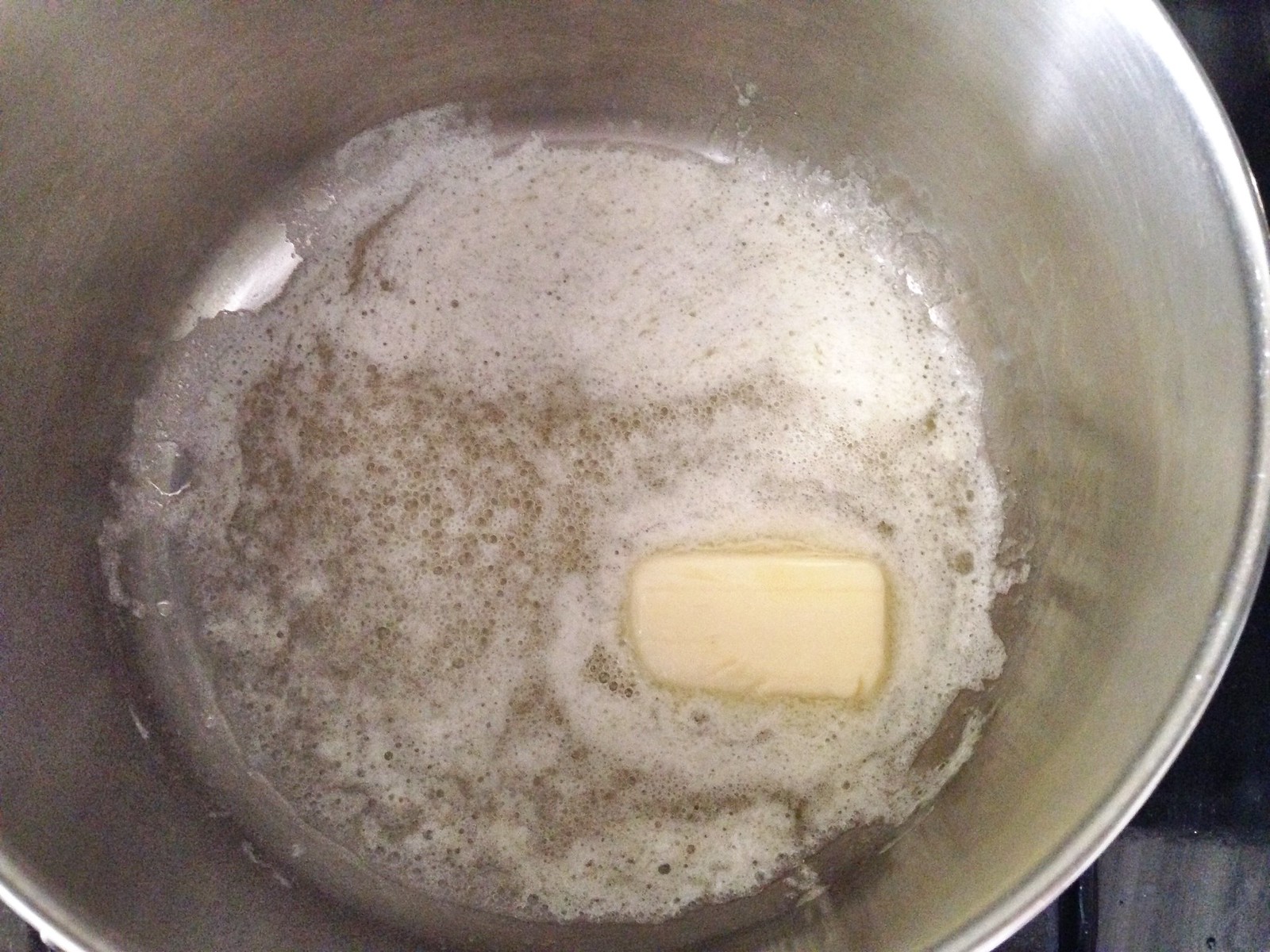A close-up photograph captures a gray-silver wok, almost entirely filling the frame, with light reflecting off its surface. Melting butter dominates the bottom of the wok, featuring a prominent yellow, rectangular pat that is partially melted. The butter appears frothy, with white and yellow bubbles, and some areas show a brown tint, indicating initial browning stages. Behind the wok, blurry, indistinct black or gray elements can be partially seen in the corners. Light from the top right accentuates the texture of the foamy, bubbling butter.